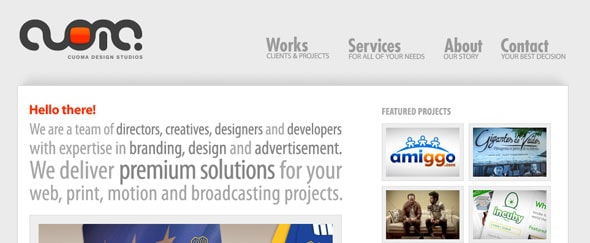The image appears to be a partial screenshot of the top section of a website, primarily focusing on the upper left-hand corner. The screenshot captures a gray banner running horizontally across the top, which is segmented by a thinner gray strip extending to the right and left, abruptly cut off at the edges, indicating it is incomplete.

On the top left of the gray banner, there is a company logo that consists of a black, snake-like line stretching across the middle, along with a circular element filled with red and some small, unreadable text below it. To the right of the logo within the gray banner, four navigation links are displayed: "Work," "Services," "About," and "Contact," each accompanied by small, descriptive text underneath.

Beneath this banner on the left side is a white box containing red text that reads "Hello there!" Below this greeting, there is gray text that varies in size and boldness, explaining, "We are a team of directors, creators, designers..." providing a brief introduction to the team.

To the right of the introductory text, there's a section titled "Featured Projects," in small gray text. Below this heading, four images are arranged in a grid (two on top and two on the bottom), likely representing clickable project links for more information. The bottom portions of these images are cut off in the screenshot.